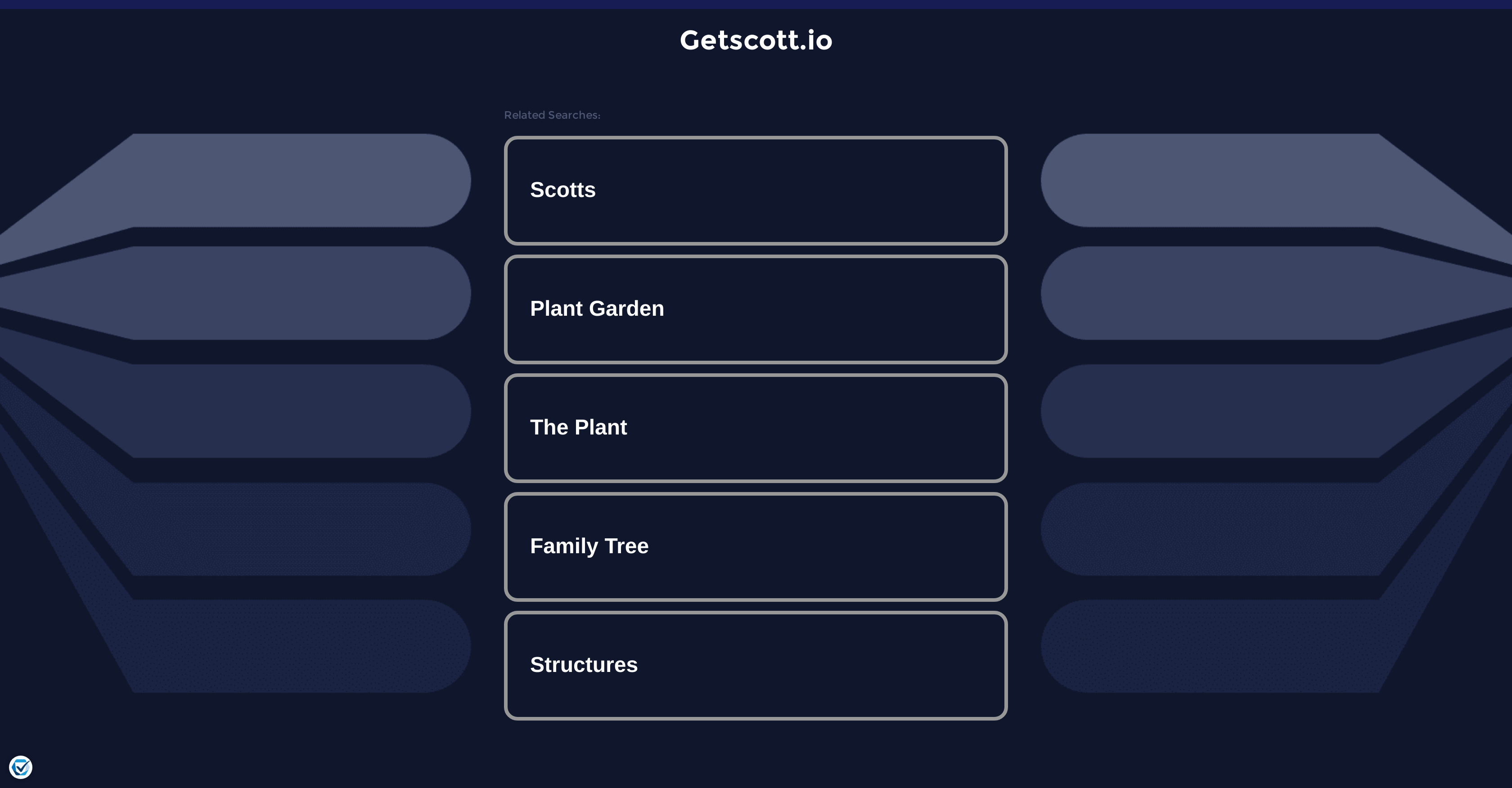This image showcases a visually structured webpage with a dark blue background and contrasting white text. Prominently centered at the top, the text "getscot.io" indicates the URL of the page. Below the main header, a section titled "Related Searches" features five distinct search terms, each framed by a grey outline. These searches include:

1. Scots
2. Plant Garden
3. The Plant
4. Family Tree
5. Structures

Each search term appears in white text with a uniform grey border.

Flanking the search terms are graphical bars. These bars, ten in total, are evenly split with five on the left and five on the right of the searches. The bars exhibit a gradient transition from blue at the top to dark blue at the bottom. On the left, the bars extend to the left side and on the right, they extend to the right side. Their size diminishes progressively as they move away from the center.

In the bottom left corner of the image, there is a white section containing an element highlighted in blue with a dark blue check mark, adding a contrasting focus point.

Overall, the page layout is methodically organized with color gradients and symmetrical bar designs enhancing the visual appeal and readability.